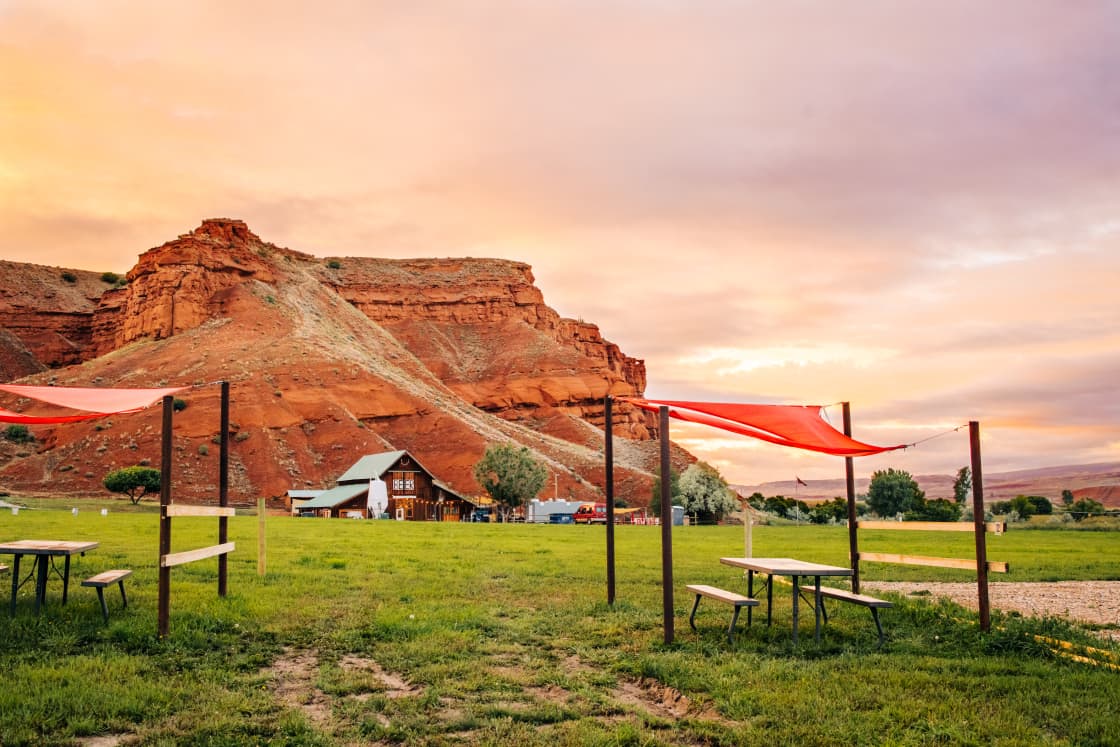In this photograph taken during dusk, hues of pink, purple, and gray paint the sky as the sun sets behind clouds. Central to the image are two white, old-fashioned picnic tables, each sheltered by vibrant red awnings, which are tied at the corners to brown wooden poles, providing shade. These are situated on a green grassy area, with some patches worn. Behind the picnic tables stands a brown house with a distinctive white roof, possibly a farmhouse, rest stop, or a lodge. The background is dominated by a massive red rock formation, casting a striking contrast with the surrounding foliage of trees and bushes. A light wooden fence runs through the scenery, and a red flag can be seen further in the distance, adding to the rustic charm of this picturesque outdoor setting.